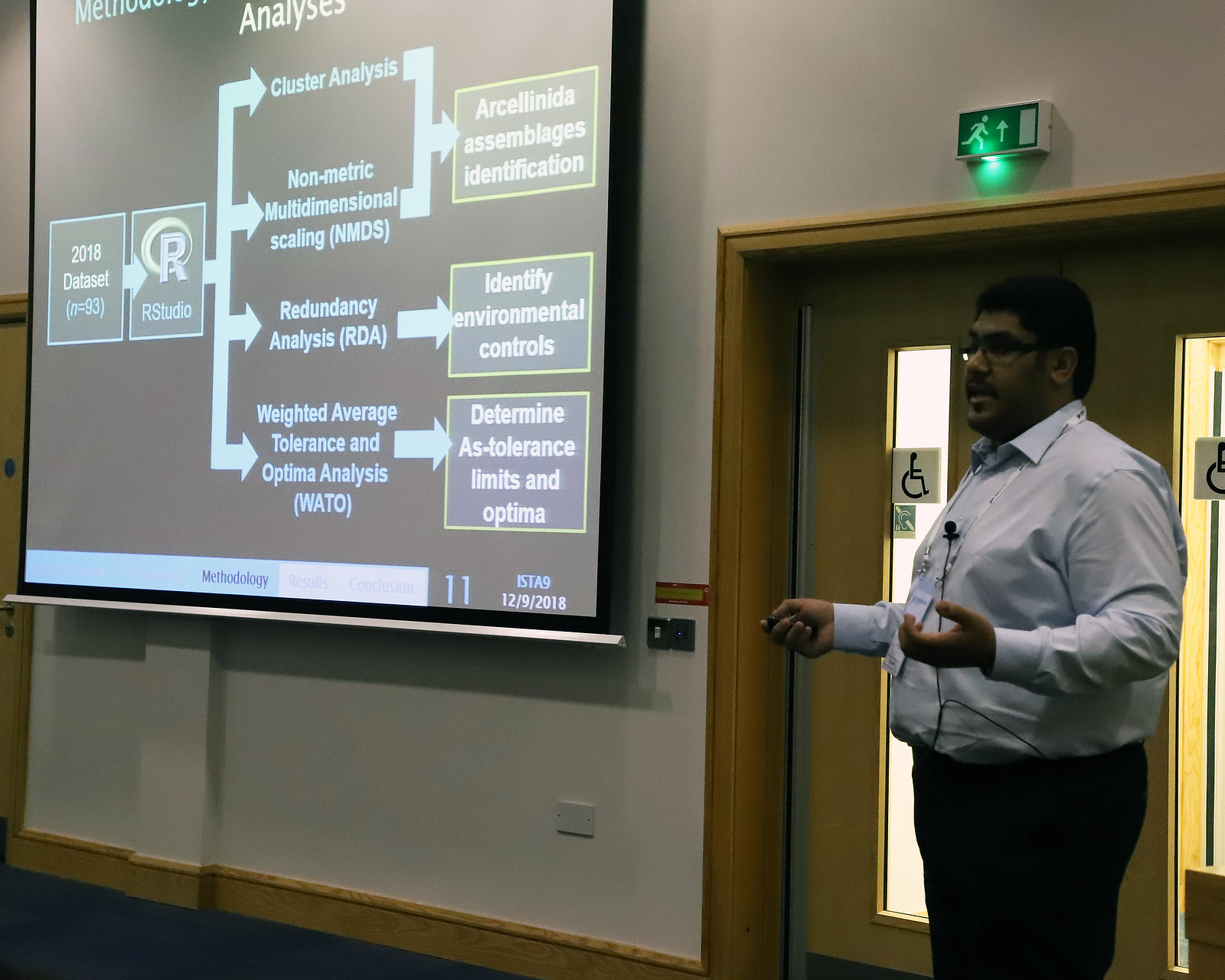In this image, we see a man, likely of Indian descent, standing in front of a set of brown doors with a green lit-up exit sign above them. He is slightly overweight and is wearing a light blue collared shirt along with black pants, and has dark brown hair. Attached to his shirt is a microphone, indicating that he is giving a presentation. In his hand is a clicker with buttons, which he seems to be using to interact with a large pull-down screen on the wall in front of him. The screen displays a detailed presentation that includes topics such as "2018 Data Set," "RStudio," "Cluster Analysis," "Non-Metric Multidimensional Scaling (NMDS)," "Redundancy Analysis (RDA)," and "Weighted Average Tolerance and Optimum Analysis (WATO)." The image appears to capture an indoor setting, likely during the day, where the man is discussing technical or educational content. The overall color palette includes blue, brown, white, green, yellow, and gray. A carpeted floor is visible, and a ceiling-mounted projector is shining onto the screen.